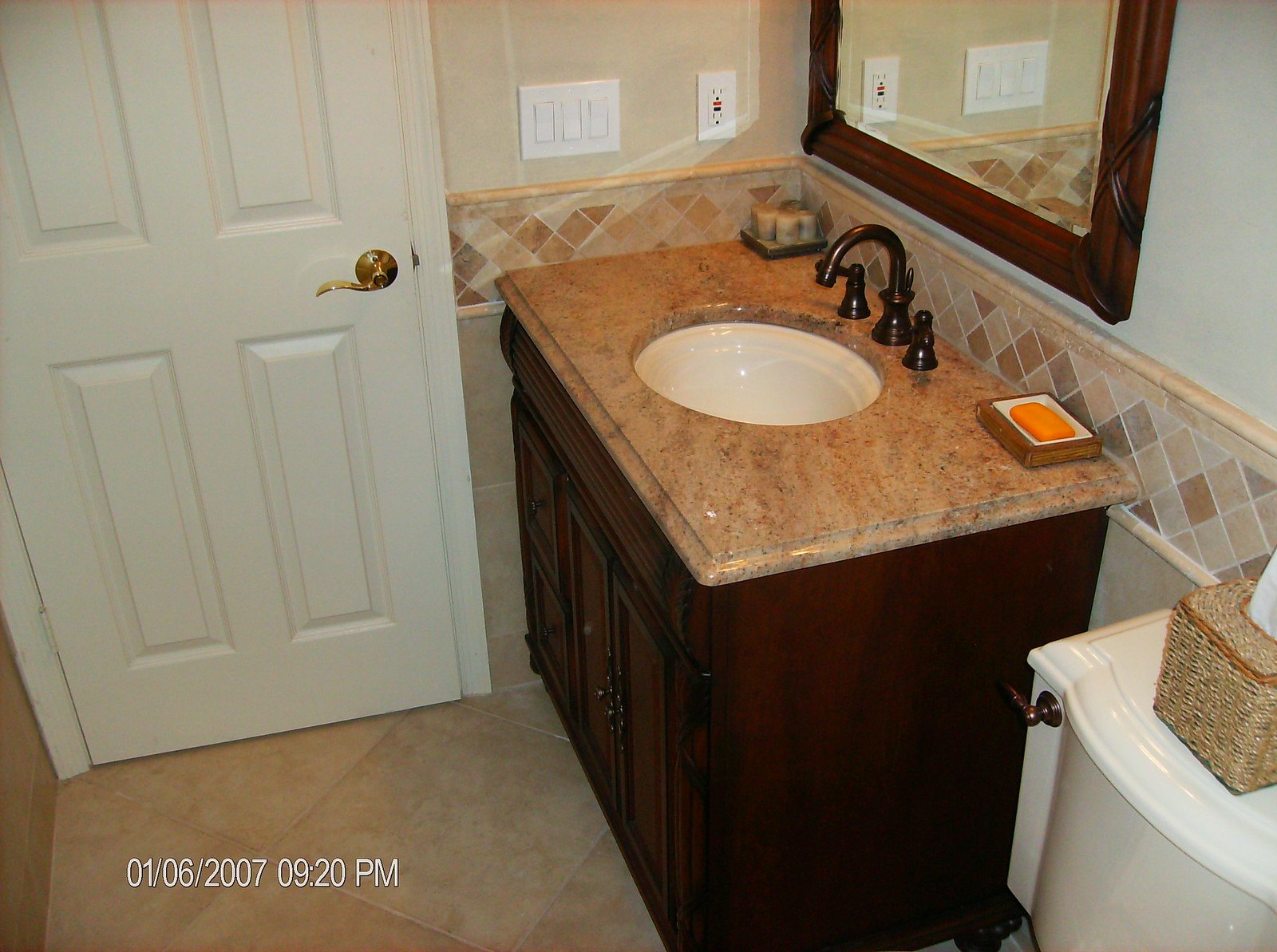The photo captures a well-organized bathroom area with various elements in detailed view. On the left, a white door featuring four rectangular indentations is equipped with a gold doorknob and a long gold handle. Moving right, the wall hosts a set of push-button light switches and a white electrical outlet. Adjacently, a mirror bordered by dark brown wood hangs prominently.

Below the mirror, the sink area boasts a brown faucet flanked by two smaller knobs. A brown soap dish holding orange soap rests on the white deep sink. Underneath, very dark brown cabinets provide storage space. To the right, the top of a toilet is visible, featuring a brown handle and a woven brown tissue holder with white tissues peeking out.

The bathroom floor consists of large brown tiles, creating a cohesive look. In the lower left corner of the image, white text indicating the date and time reads "01/06/2007 09:20 PM."